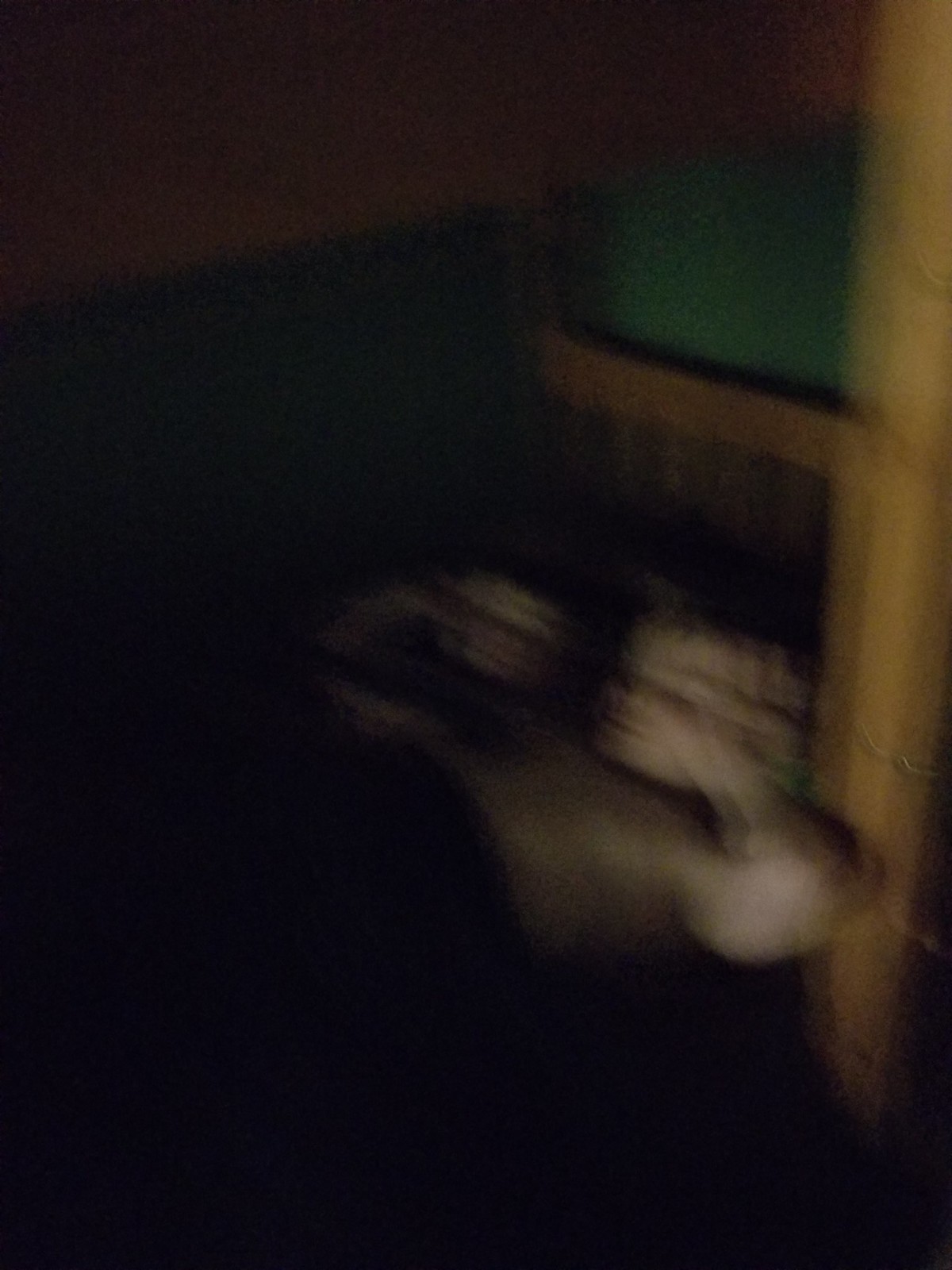This image is a blurry, rectangular photograph primarily featuring a young boy lying down, possibly on a bed or couch. The boy, who appears to be white-skinned and shirtless, has his left hand positioned near his head, almost as if he is flexing his biceps. His body from around the mid-stomach downwards is obscured by a blanket or some other covering. The image, taken quickly and in motion, leaves much of the scene in shadow, especially on the lower left side which appears completely black. On the right side, there is a wooden frame, likely part of a bed structure, suggesting the possibility of a bunk bed. Additionally, there is a green object in the background and the back wall has an orange hue. The overall darkness and distortion of the image make it challenging to discern finer details.